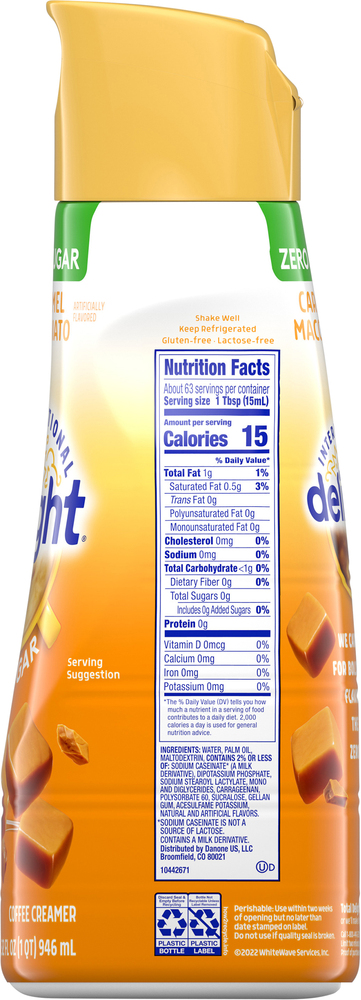The image depicts the side of a bottle of International Delight Caramel Macchiato Zero Sugar Coffee Creamer, featuring a detailed nutrition facts label. The bottle design includes a gold plastic cap, a green band at the top reading "zero sugar," and a white background adorned with gold lettering for "caramel macchiato." The nutrition facts label, in blue lettering against the white background, states 63 servings per container, with each serving being one tablespoon (15 milliliters). Each serving contains 15 calories, 1 gram of total fat (including 0.5 grams of saturated fat and 0 grams of trans, polyunsaturated, and monounsaturated fats), zero grams of cholesterol, sodium, total carbohydrates (with zero dietary fiber and sugars), and protein. The label also indicates that the product is gluten-free and lactose-free, and should be shaken well and kept refrigerated. Additionally, you can see the bottle’s recycling information and decorative squares of caramel near the bottom right corner, along with the words "coffee creamer." The image focuses solely on the side of the bottle, capturing all the pertinent nutritional and ingredient details.